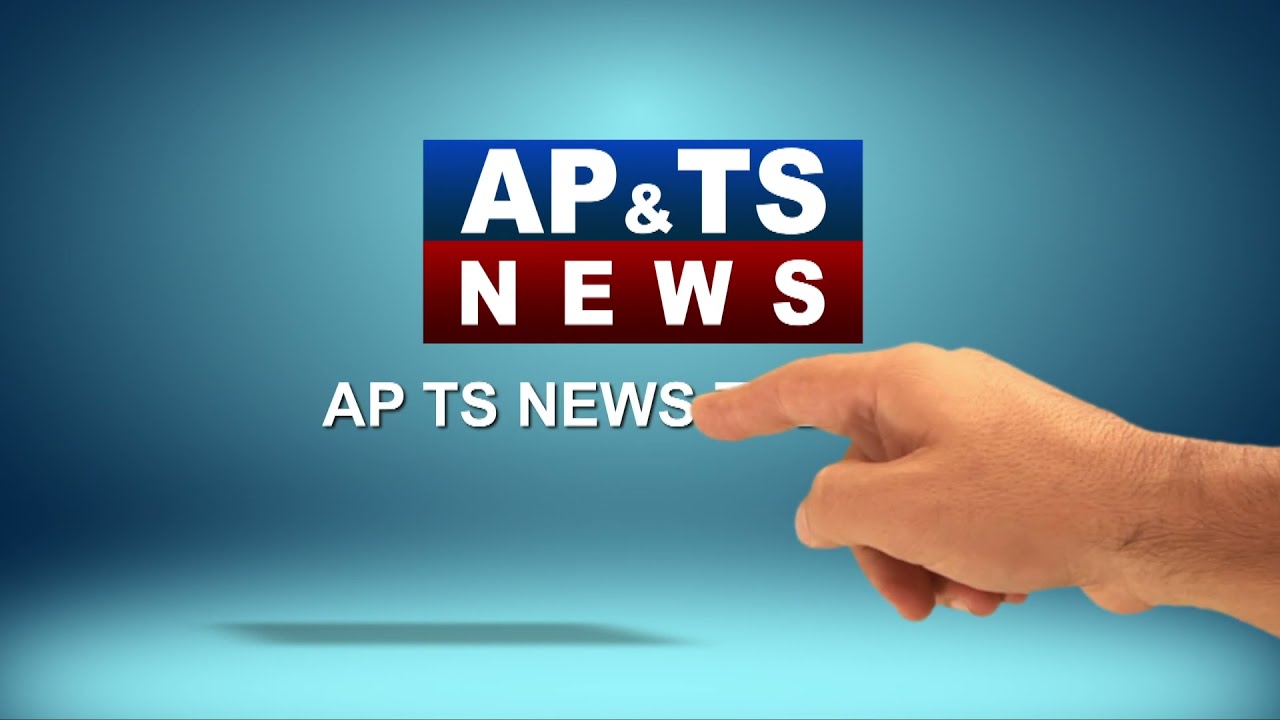The image features a color photograph with a blue background that transitions from light teal in the middle to darker shades towards the edges. Central to the image, there's a rectangular logo divided horizontally with a top blue section and a bottom red section. In the blue area, white capital letters spell out "AP" and "TS," while "NEWS" is displayed in the red section. Below the rectangular logo, additional white block text states "APTS NEWS," though part of this text is partially obscured by a hand. The hand, light-skinned and slightly hairy, appears to be a right hand pointing at the text, with the finger covering additional letters. The background includes shadowed areas adding depth to the image, and the text itself casts a grey shadow underneath it.